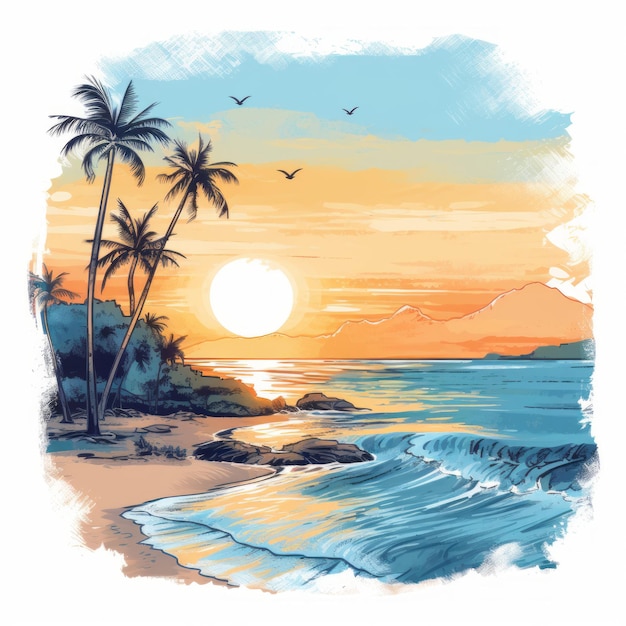The artwork is an intricate illustration of a tropical beach at sunset. On the lower left, a sandy beach decorated with several palm trees and rocks extends towards a serene body of water on the right, where gentle waves lap onto the shore. Adding depth to the image, a variety of vegetation clusters near the upper part of the beach, including some prominent green cliffs. 

In the midsection, the calm sea captures the reflection of a bright, white-yellow sun, positioned slightly to the left, setting behind a range of mountains that rise and expand towards the right. The sky is a blend of vibrant colors: the lower part glows with golden-orange hues from the sunset, while the upper part remains a tranquil blue, dotted with a few white clouds. The scene is completed by three birds soaring gracefully above, enhancing the picturesque and serene quality of the beach landscape. The entire image has rough, smudged edges, creating a unique, somewhat softened frame around the vibrant depiction of this tropical paradise.